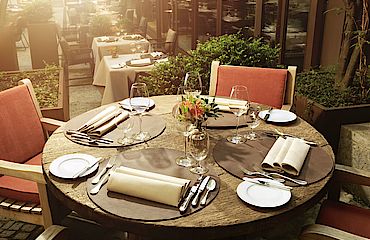The image is a color daylight photograph capturing an outdoor dining area at a restaurant, bathed in bright sunlight streaming in from the upper left. The focus is on a small, round, wooden table set for four people. Each place setting features a large circular brown placemat, topped with a cloth napkin and an array of silverware: two forks on the left, two knives and a spoon on the right. Additionally, there is a small white plate with a knife laid across it, and both a wine glass and a water glass at each seat. The table centerpiece is adorned with a flower arrangement, adding a touch of natural beauty. Surrounding the table are four wooden chairs, each with a reddish cushion; however, the two nearest to the viewer are partially obscured. In the background, there are more square tables, some set for pairs and covered with tablecloths, arranged alongside planters filled with plants and possibly a tree on the right. Beyond these tables, a row of windows line a brown wall, reinforcing the outdoor ambiance of this dining space.